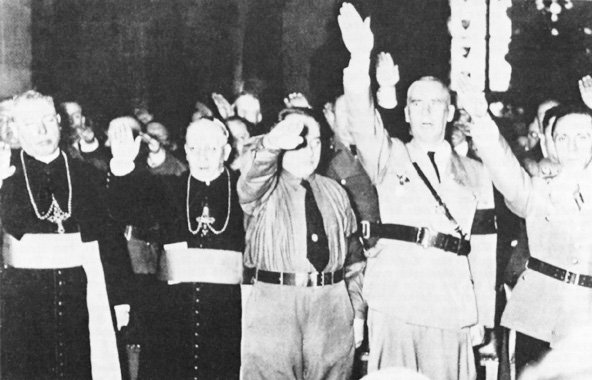This is a black and white photograph, likely from the World War II era, depicting an outdoor scene. The image is slightly faded but shows a group of men facing the camera, all performing the infamous Nazi salute with their arms raised. On the left, two men are dressed in religious garb, wearing long dark robes, white sashes around their waists, and large crosses hanging down to their chests. In the center, an older man in high-waisted light-colored pants and a dark tie also has his arm raised. Flanking him, two tall men are dressed in light-colored military uniforms with dark ties and belts, each performing the salute. Behind these central figures, more individuals can be seen, also raising their arms. They stand in front of an indistinguishable building, and the photograph suggests it is daytime. The overall impression is of a significant historical moment captured on film.